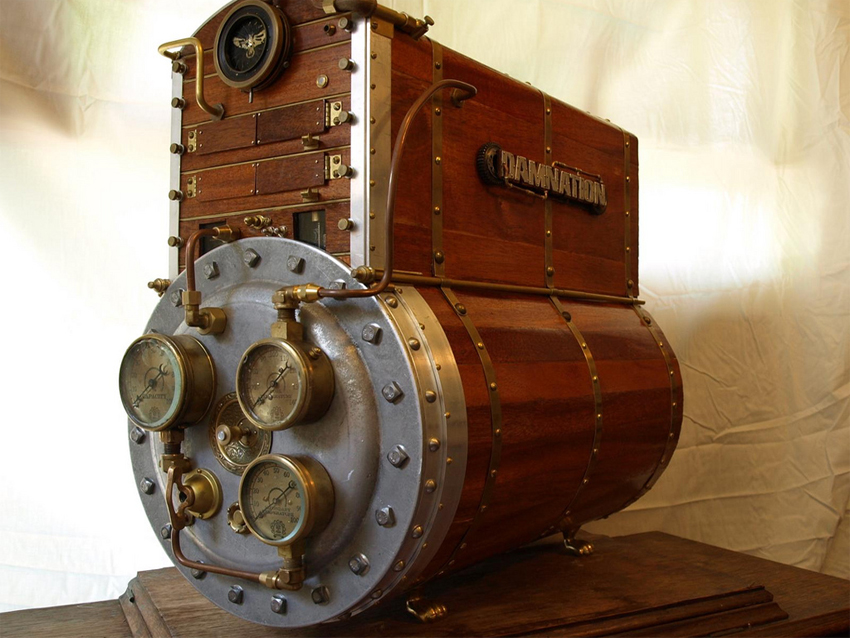This photograph captures a vintage device that exudes an air of mystery and historical intrigue. The device's foundation is a cylindrical base resembling a red or maroon-red barrel, adorned with a silver metal cap secured by screws on its larger, left-facing end. This base features three brass gauges, each with needles poised at zero, which are mounted on a round metal panel held by numerous bolts and rivets against a folded metal outer ring. Attached to or emanating from the top edges of these gauges are copper pipes bending upwards and merging into the structure above.

Resting on this cylindrical base is a horizontally aligned rectangular box crafted from dark oak-like wood, bordered with silver metal edgings and fastened with screws. The box has a distinctive peaked top and is uniformly trimmed. At the very top of this peak, there's a circular emblem poised like a gauge, featuring an eagle with outspread wings against a black background. Additionally, a metallic badge on the side of the box proudly displays the word "Damnation" in silver letters, though some letters appear less legible due to the angle of view.

Supporting the cylindrical base are brass feet that keep it balanced on a wooden block, further stabilizing the device on what appears to be a display table. The entire setup is set against an aged, yellowy white backdrop, contributing to the vintage and timeless aura of this enigmatic apparatus.